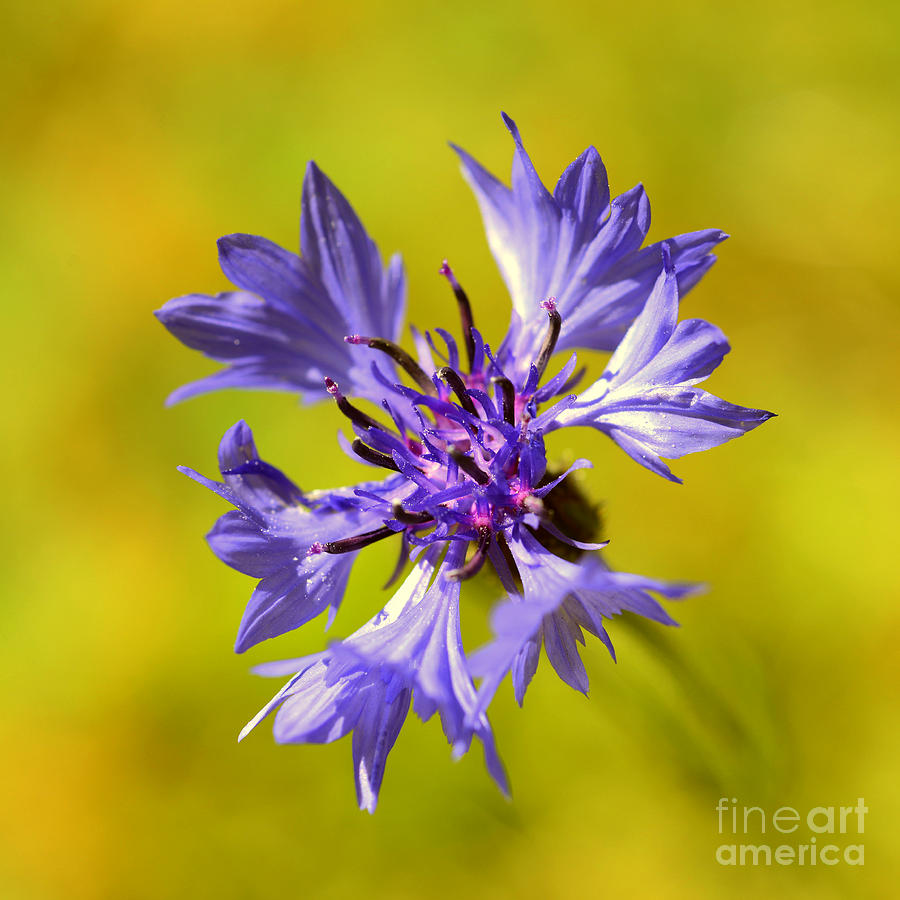This image captures a stunning close-up of a large purple flower set against a blurred yellow and green background, creating a vivid contrast that makes the flower stand out. The background, reminiscent of split pea soup with its blotched yellow and green hues, is so blurred that the flower’s stem seems to blend into it, drawing all focus to the flower itself. In the bottom right corner, the image bears a "Fine Art America" watermark, hinting that this is a piece of artwork, likely a poster or print.

The flower, striking in its violet purple shade, features six prominent petals or blossoms radiating from its center. Each petal is open and extends outward, with dew drops and pollen crystals adding a touch of realism to the image. The center of the flower is intricate, with pink and crystalline structures where the pollen pods are located, some even appearing to release pollen into the air. The detailed appendages in the middle, varying in height and direction, further enhance the flower's exotic and tropical appearance. This highly detailed photograph showcases the flower in such magnification that its delicate textures and vibrant colors are exquisitely highlighted.